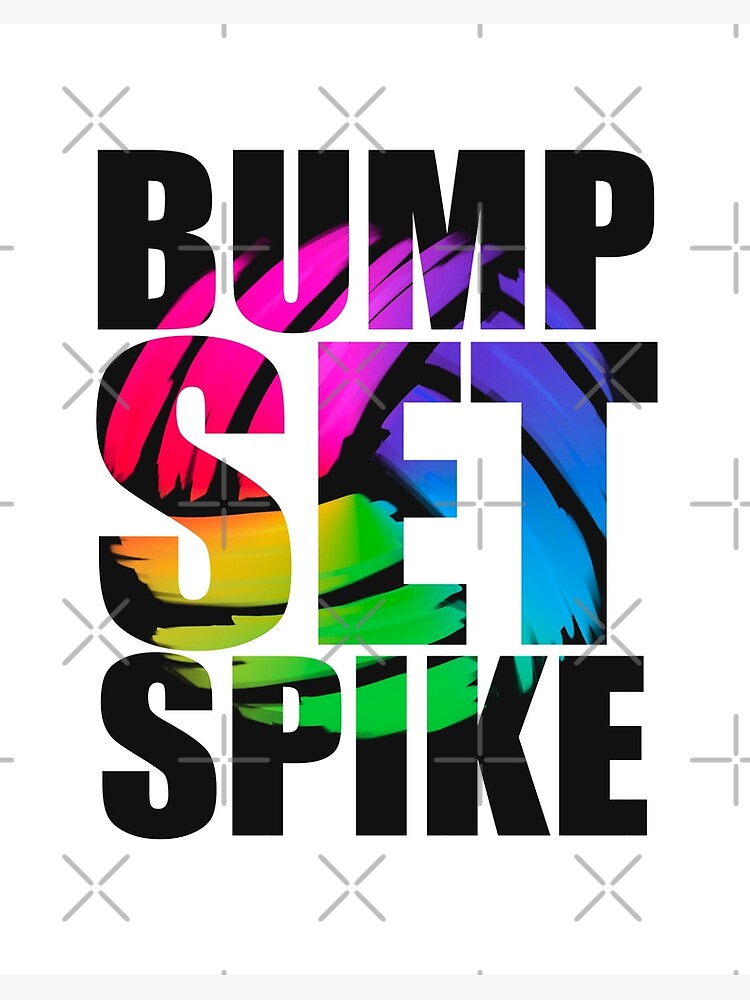The image features a logo on a pure white background adorned with a pattern of disjointed X's, resembling watermarks, scattered throughout the design. Dominating the center of the image is bold, capitalized text in black that reads "BUMP, SET, SPIKE," referring to the sport of volleyball. "BUMP" and "SPIKE" are of similar height and font, while "SET," positioned in the middle, is significantly larger. Embedded creatively within the text is a vibrant volleyball illustration. This volleyball, depicted in a cartoonish style, features three-stripe segments of rich colors: pink, red, orange, green, blue, and a hint of purple. Although incomplete, with its top in pink, bottom in green, and right side in blue and purple, the design cleverly conveys the essence of a volleyball. Overall, the image combines dynamic text with colorful artistic elements to highlight the theme of volleyball.